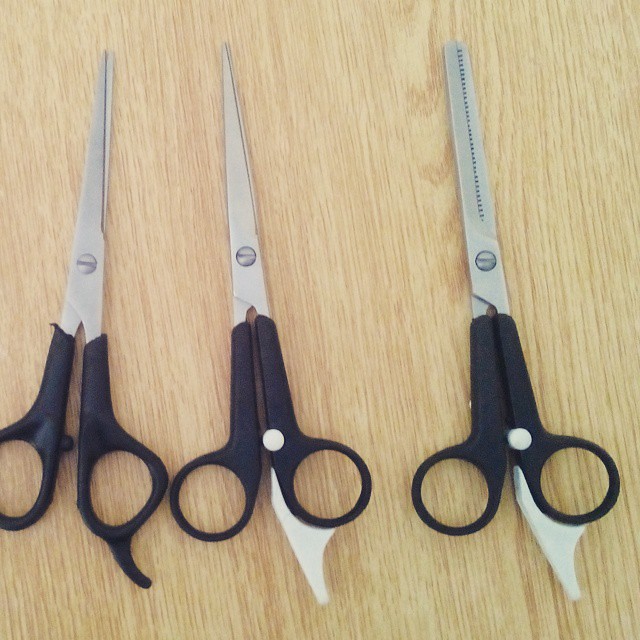In this well-lit image, three pairs of professional barber scissors are arranged on a light brown wooden table, which features darker brown lines and grains. Each scissor has handles with black rubber grips and additional ergonomic features. On the left, the first pair of scissors has a traditionally sharp, silver steel blade and a black finger rest protruding from one of its loops. The middle pair of scissors is similar but includes a white finger rest and a small white dot between the handles for added comfort and precision. Both pairs are sleek and pointed, ideal for precise cutting. On the right side is a pair of thinning shears, recognizable by their serrated, sawtooth blade designed for thinning thick hair. This pair also has a black handle with a white finger rest integrated into one of its loops, similar to the middle scissors. The high level of detail and the bright overhead lighting make the tools easy to distinguish in the photograph.